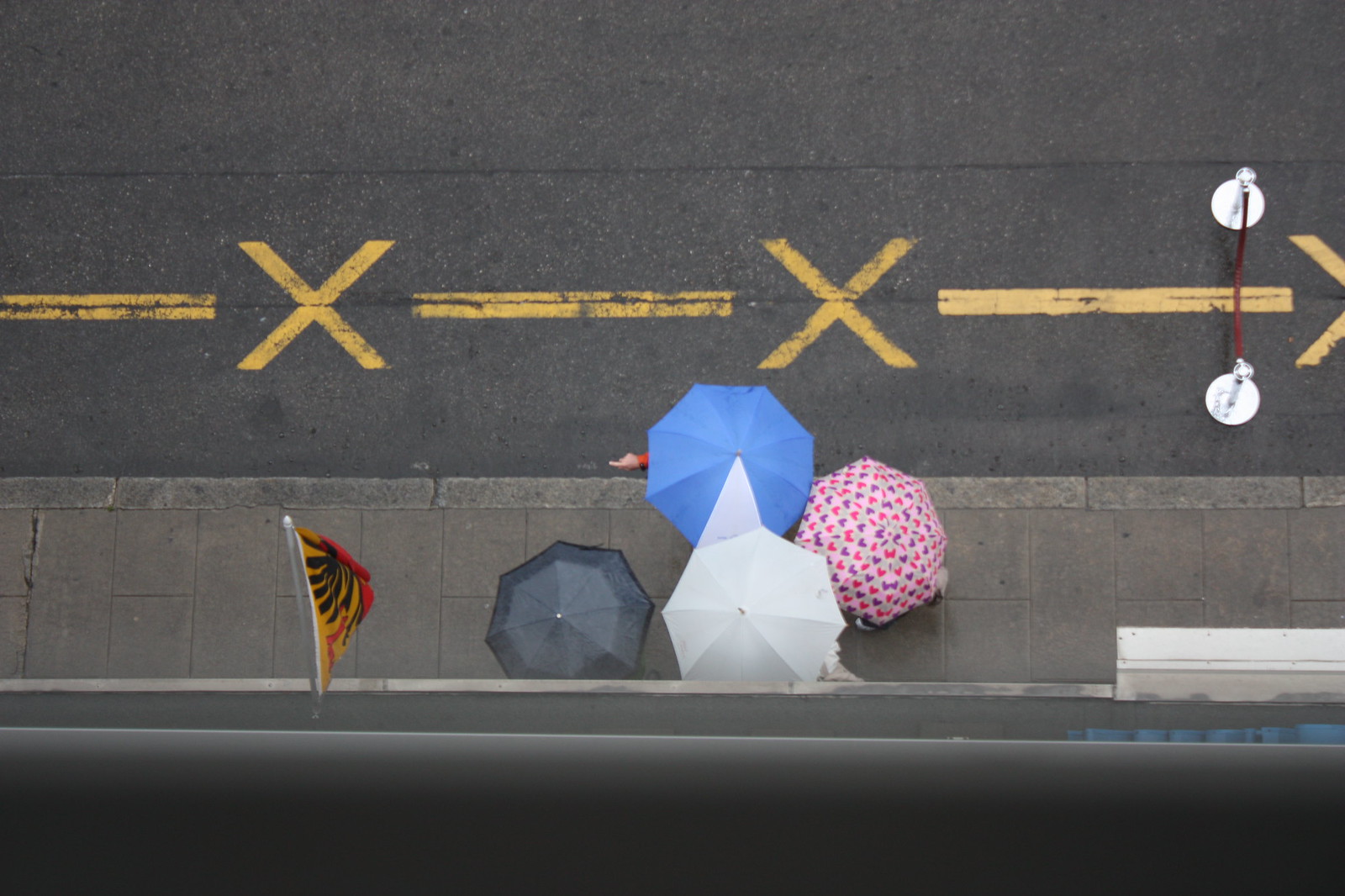This image captures a rainy street scene through an overhead perspective, likely taken from a window in a building above the sidewalk. Four people under open umbrellas are visible, with the umbrellas colored black, blue, white, and pink with dark pink and purple hearts. The street features yellow dashed lines and X markings, suggesting parking restrictions or a bike lane. The wet appearance of both the street and sidewalk, composed of gray-tiled concrete, confirms recent rainfall, though no raindrops are visible. A flag, yellow and orange in color, is hanging downward from a nearby building, adding a touch of vibrancy to the subdued, rainy atmosphere. Additionally, a hand is seen sticking out from under one of the umbrellas, pointing left. The shot includes various road signs, barriers, and possibly parking signs reinforcing the urban setting.